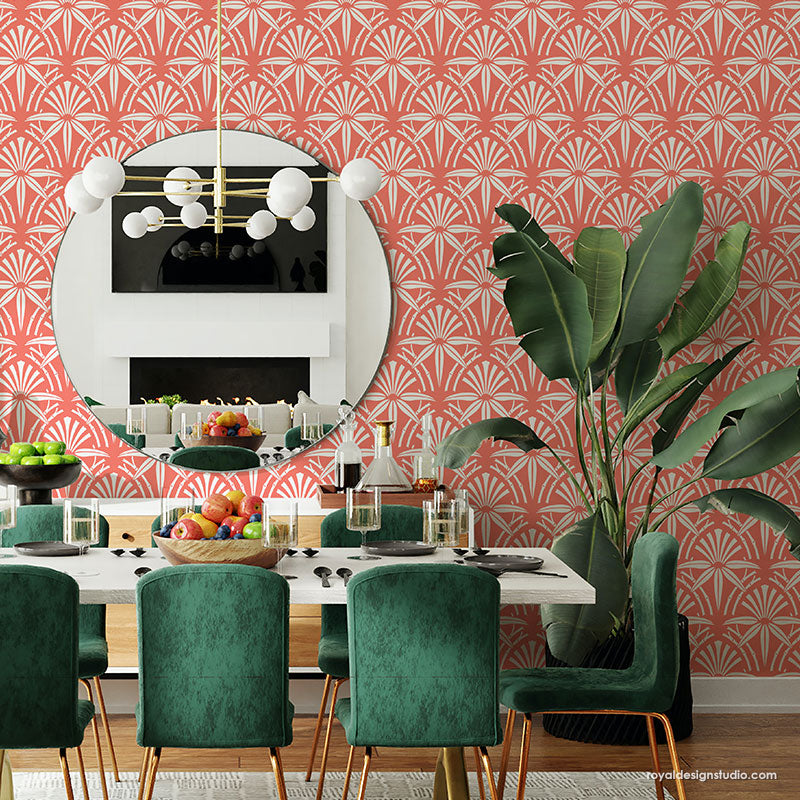The dining room is a vibrant and modern space characterized by its tropical and colorful design elements. The focal point is a long white table surrounded by at least six green velvet chairs with wooden or copper-toned metallic legs. Each chair is set with a grey plate, silverware, and a glass, exuding a sense of organization and elegance. The table's centerpiece is a bowl of assorted fruits, including apples and grapes, adding a fresh and lively touch to the setting.

The room features a salmon-colored wallpaper adorned with a floral pattern, possibly hibiscus, which echoes the tropical theme. On the back wall, a large round mirror reflects the room's details, including a modern chandelier. A substantial rubber tree in a black planter stands prominently, complemented by the wallpaper's design. Additional tropical elements include a bird-of-paradise plant also placed against the back wall.

Adding to the intricate details are a few jars containing various liquids on a side table, further enriching the room's texture. The design is attributed to yourdesignstudio.com, indicating a thoughtful and curated approach to modern, artsy dining room decor.